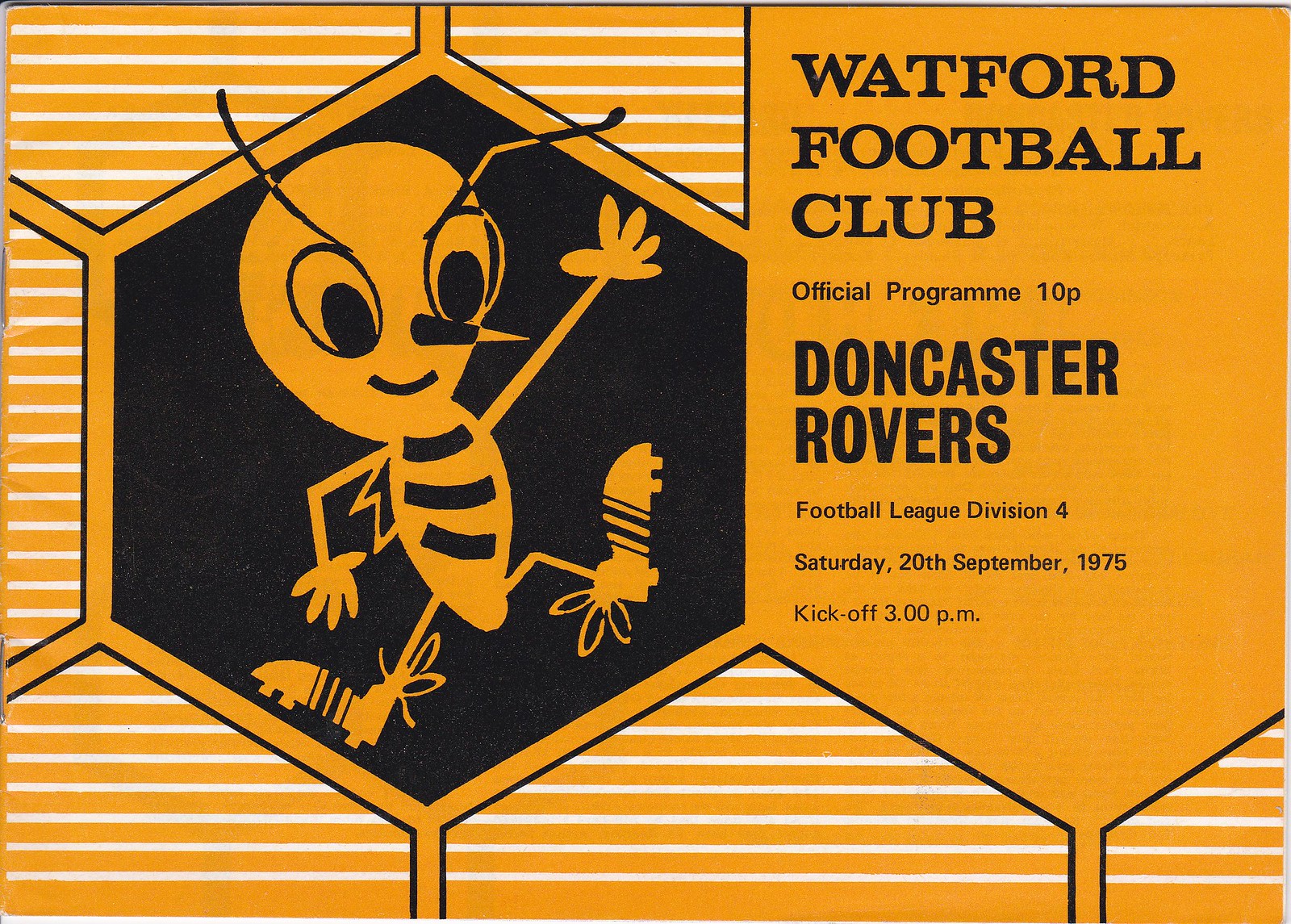The image features the front cover of an official program for a soccer match, set against an orange background. Black text prominently declares "Watford Football Club, Official Program, Doncaster Rovers, Football League, Division IV," with specifics including "Saturday, 20th of September, 1975," and "kickoff at 3 o'clock." To the left, there is an illustration of a small bug, possibly a bee, wearing soccer cleats. The text is situated to the right, while the bug logo is positioned to the left. The overall design suggests it is a program cover handed to attendees at a soccer game, radiating a nostalgic 1970s aesthetic with its color palette and layout.